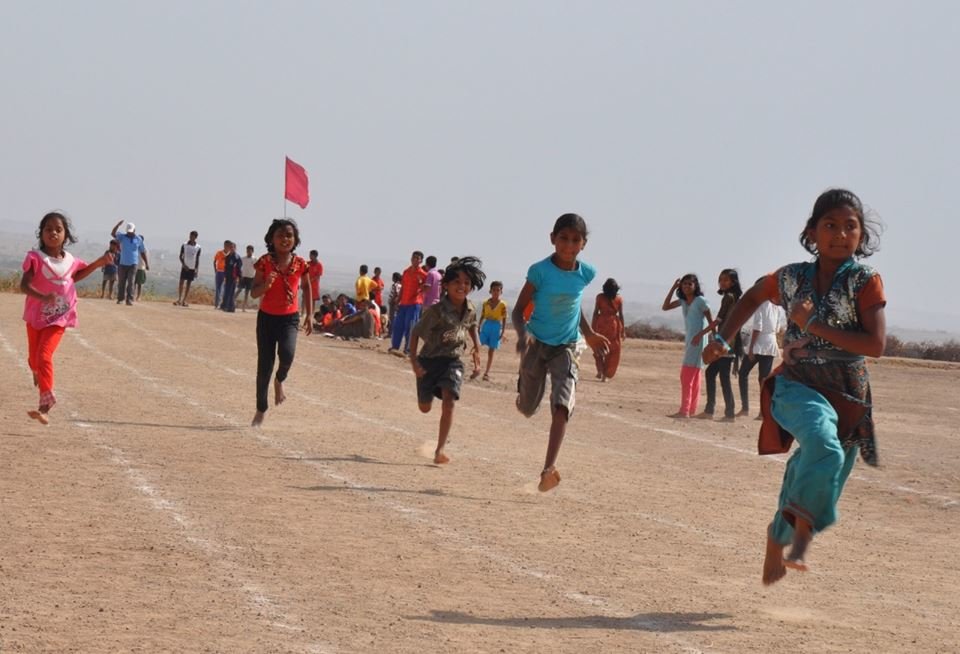In the foreground of this outdoor daylight photograph, a group of five young children—four girls and one boy, all appearing to be barefoot and possibly of Indian descent—are racing along a dirt track marked with white lines. The track seems to be situated in a barren or desert-like area. Leading the race is a girl dressed in authentic garb, followed closely by a girl in a blue shirt and gray shorts. Trailing behind them is a boy wearing gray pants and a brown shirt, followed by a girl in a red shirt and long pants, with the final runner being a girl in pink and red pants. The children are captured in mid-stride, some seemingly floating above the ground due to their speed. The background reveals an enthusiastic crowd of parents and onlookers, cheering the racers on. The sky is a bright but slightly overcast blue, and the scene is further illuminated by sunlight coming in from the right side of the image. Additionally, there is a red flag visible in the background along with a hazy view of what could be a town, adding to the lively atmosphere of the event.